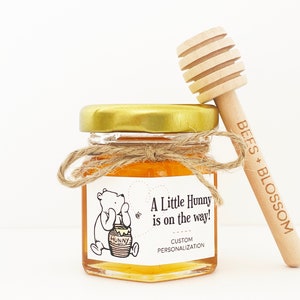This image features a small, six-sided glass jar of honey, adorned with a golden-colored twist-off lid and a bow made of brown twine wrapped around the top. The jar is elegantly presented on a clean, white background. A white label is affixed to the front of the jar, featuring an illustration reminiscent of Winnie the Pooh sitting beside a bucket of honey. The label bears the words "A little honey is on the way" in black, with the option for custom personalization indicated below. Accompanying the jar is a wooden honey wand, engraved with the phrase "Bees Plus Blossom," leaning against the right side of the jar. This product appears to be a customizable gift item, possibly ideal for events such as weddings to give guests as a thank you gift.